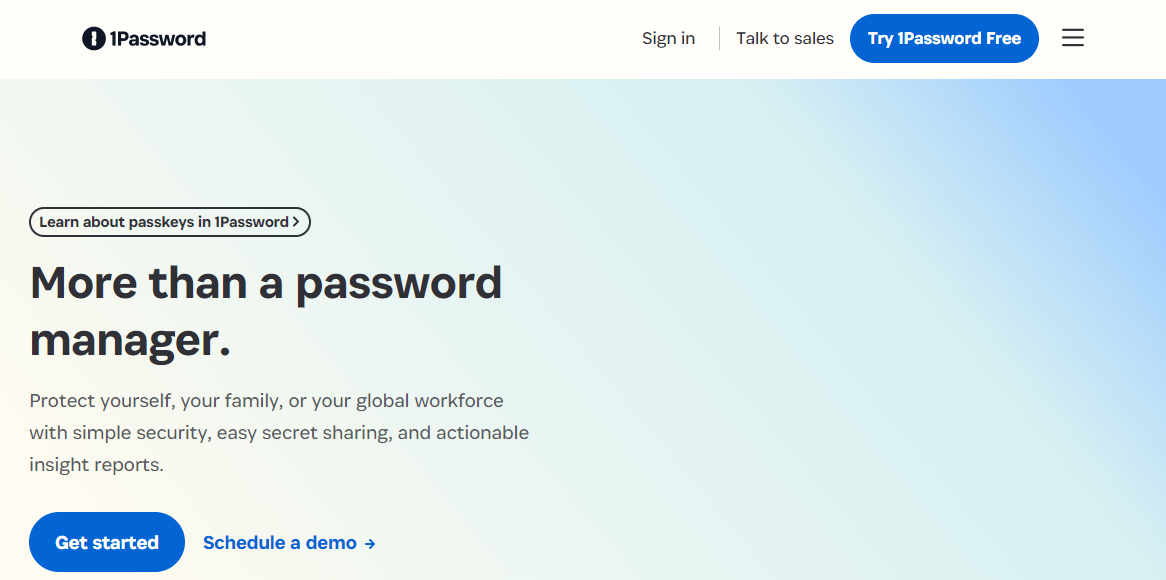A promotional image featuring a blue gradient background that transitions from a very light gray on the left to a medium tone blue on the right. The image prominently displays several call-to-action buttons and text. At the top, there is a white oval button with the text "Sign In," a button labeled "Talk to Sales," and another inviting users to "Try 1Password Free" inside a blue oval. 

In the top-left corner, a hamburger icon suggests a menu. Below, a headline reads "Learn About Passkeys in 1Password" accompanied by a right arrow icon. 

Further down, a tagline emphasizes the comprehensive security offerings: "More than a Password Manager." The text elaborates, "Protect yourself, your family, or your global workforce with simple security, easy secret sharing, and actionable insight reports."

At the bottom of the image, a blue rectangle button with the text "Get Started" in white is displayed prominently. Next to it, in blue text, is a "Schedule a Demo" link, also accompanied by a right arrow icon, urging users to take the next step.